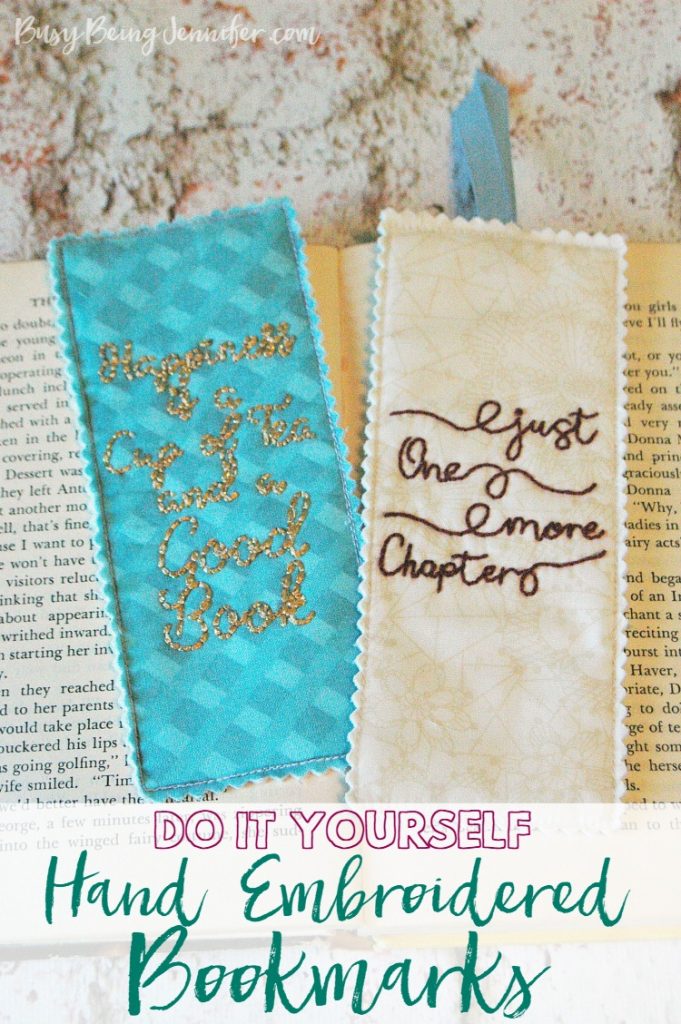The image showcases a photorealistic, beautifully detailed scene, filling the top two-thirds with a photograph of an open book, showing both left and right pages laden with black text on white paper. Resting gracefully atop the open book are two distinctive fabric bookmarks.

To the left, a rectangular bookmark features a turquoise felt with a striking lattice pattern, created by alternating shades of turquoise. Embroidered in gold thread at its center are the words "Happiness is a cup of tea and a good book." The design and message exude a sense of coziness and comfort.

On the right, another rectangular bookmark complements the first, crafted from white felt adorned with a subtle floral and geometric pattern in faint tan. A blue ribbon embellishes its top, while elegant brown cursive embroidery spells out "Just one more chapter," capturing the reader's endless yearning for more literary adventures.

The backdrop consists of a soft, white or beige carpeted area, adding warmth and homeliness to the scene. At the top of the image, the semi-transparent text reads "busybeingjennifer.com" in cursive, while at the bottom, within a semi-transparent border, "Do It Yourself" is displayed in a purple font with "Hand Embroidered Bookmarks" in turquoise beneath it.